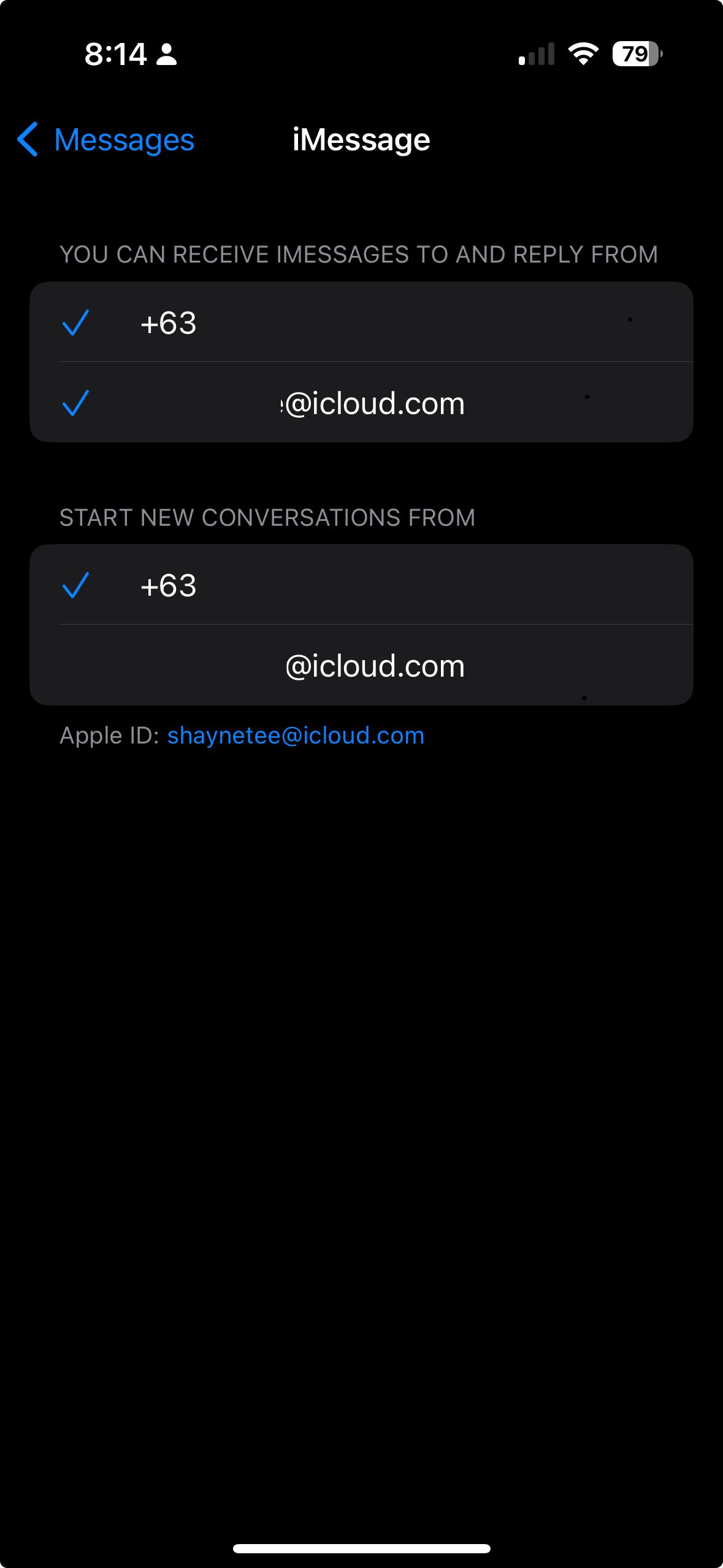The image displays a screenshot from an iPhone device. In the upper left-hand corner, the time reads 8:14, accompanied by a small icon of a person. On the upper right, the signal strength shows one out of four bars for cellular service and three out of three bars for Wi-Fi connectivity. The battery level indicator reveals that the phone was at 79% at the time the screenshot was taken. The screenshot captures a section of the iPhone's settings interface. At the top, the title "iMessage" is visible, with a blue text and arrow on the left labeled "Messages," indicating a navigation option. The highlighted section provides options related to iMessage. It reads: "You can receive iMessages to and reply from," followed by a partially obscured phone number starting with +63, and a similarly obscured iCloud email address. Another section below is titled "Start new conversations from," listing the same +63 phone number and the iCloud email address. At the bottom, the Apple ID is displayed as "shanity@icloud.com."